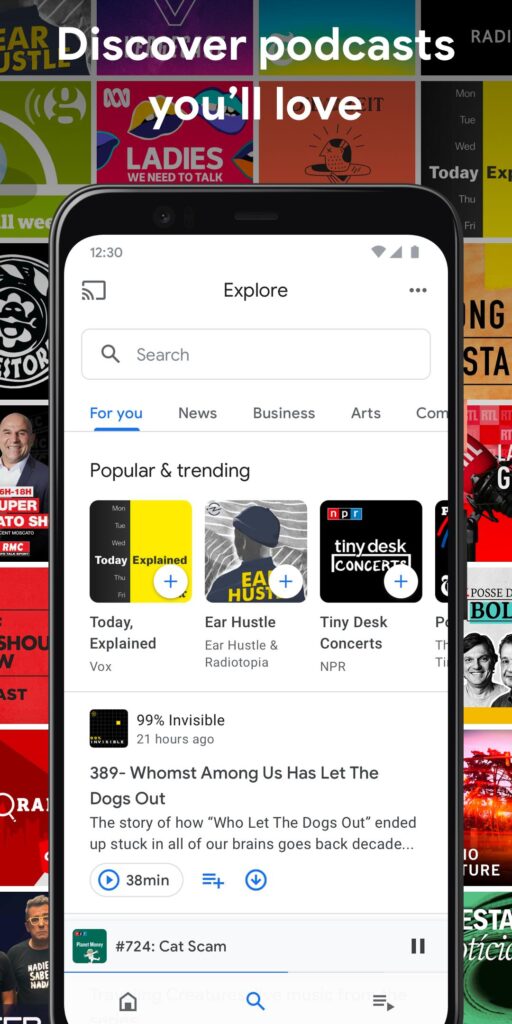The image features a tall, narrow frame with a vibrant, colorful background that resembles a comic strip, filled with an assortment of small, square images. Dominating the center is a black smartphone with a white screen. 

At the top of the image, white text reads "Discover Podcasts You'll Love." The phone’s screen displays an app interface starting with the title "Explore" and an adjacent search bar. Below this, a horizontal menu lists several categories: "For You" (highlighted), "News," "Business," "Arts," and an additional category that is partially cut off.

Featured prominently on the phone's screen is a section labeled "What's Popular and Trending," showcasing three square icons that likely represent album or podcast covers. 

Directly beneath this section is a podcast titled "99% Invisible," accompanied by some brief descriptive text. Further down, there’s another podcast entry titled "724 Cat Scam," along with a small thumbnail image to its left.

At the very bottom of the smartphone’s screen, typical app navigation buttons are visible: a home button, a search icon, and a three-bar menu icon on the right side.

Overall, the lively, colorful background frames the black smartphone, drawing attention to the detailed podcast discovery interface on its screen.